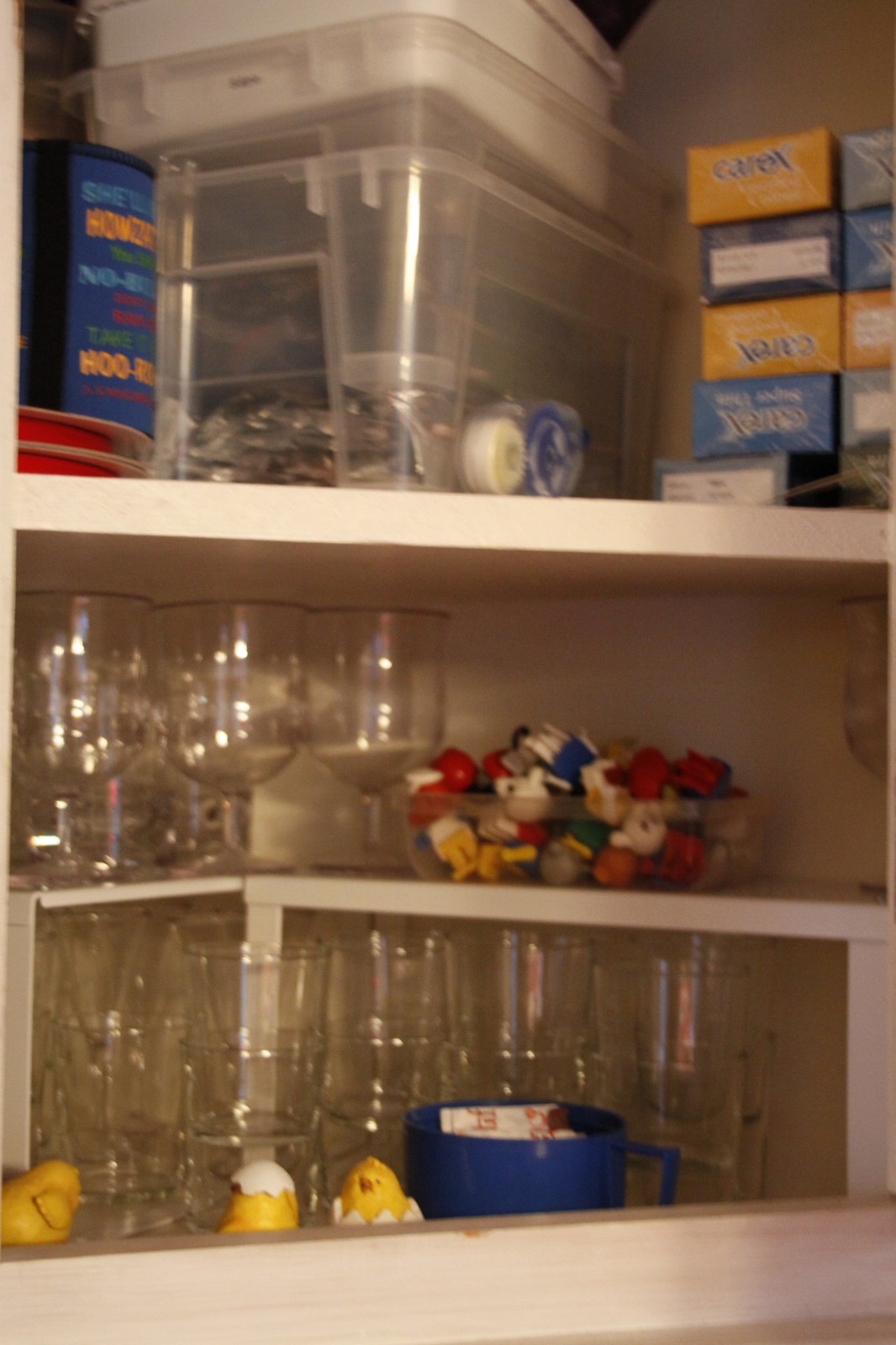The image showcases an organized pantry cabinet located above a kitchen counter. The bottom shelf prominently displays a variety of glassware, including stemware and wine goblets. Adjacent to these, there is a blue plastic cup and a collection of small figurines resembling hatching chick eggs. Additionally, there is a bowl filled with Pez candy dispensers, notable among them being dispensers with Popeye's head.

Moving to the second shelf, it primarily contains devices labeled "Carex," with the brand spelled out as C-A-R-E-X. There are several clear plastic bins; one features items wrapped in foil, identified as rolls of tape upon closer inspection. Another item on this shelf bears the marking "HOO," though further details on this item are not discernible. The Carex devices are color-coded, with approximately three yellow boxes and seven blue boxes. These blue boxes are neatly arranged in two rows of six, side by side, on the right side of the shelf. Other clear tubs and additional organized materials are also visible on this second row.